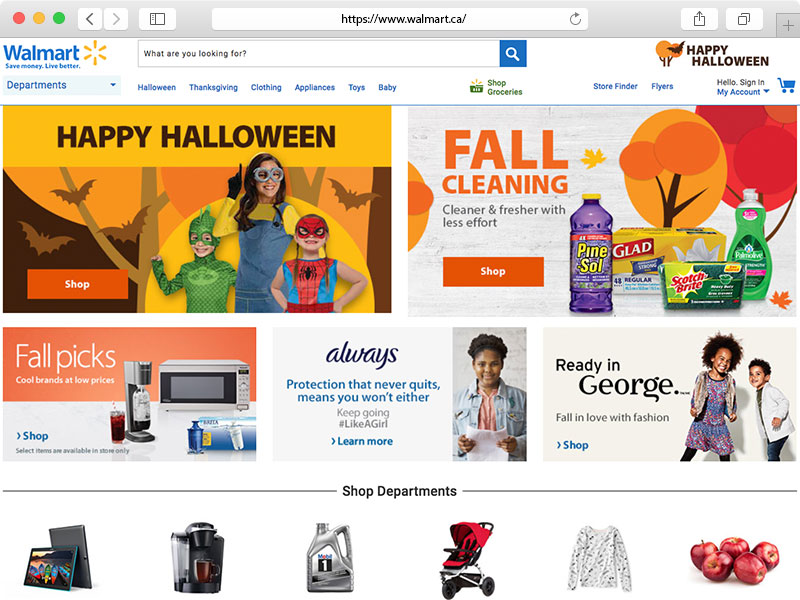The image, sourced from the Walmart website, prominently features a festive advertisement tailored for the fall and Halloween season, possibly indicating its Californian provenance given the website URL, www.walmart.ca. The left section of the ad invites viewers to a "Happy Halloween" celebration, showcasing three children joyfully clad in Halloween costumes—a Minion, Spiderman, and a green dinosaur. Below this, an orange-red rectangular "Shop" button with white lettering beckons users to explore further.

To the right of the Halloween section, the theme transitions into "Fall Cleaning," promoting the slogan "Cleaner and fresher with less effort." This area displays various cleaning supplies including Pine-Sol, Glad, Scotch-Brite, and Palmolive, set against a backdrop adorned with a sprinkle of fallen leaves and distant trees. A similarly styled "Shop" button accompanies this section, urging users to browse cleaning products.

Beneath these sections, a "Fall Picks" banner touts "cool brands at low prices." The ad further motivates with a statement about enduring protection featuring the campaign slogan, "Protection that never quits means you won't either. Keep going, #LikeAGirl. Learn more." Adjacent to this, fashion enthusiasts are prompted to "Fall in love with fashion" under the "Ready and George" tagline. Lastly, a navigational prompt to "Shop Departments" and additional clickable areas are provided at the bottom for comprehensive browsing.